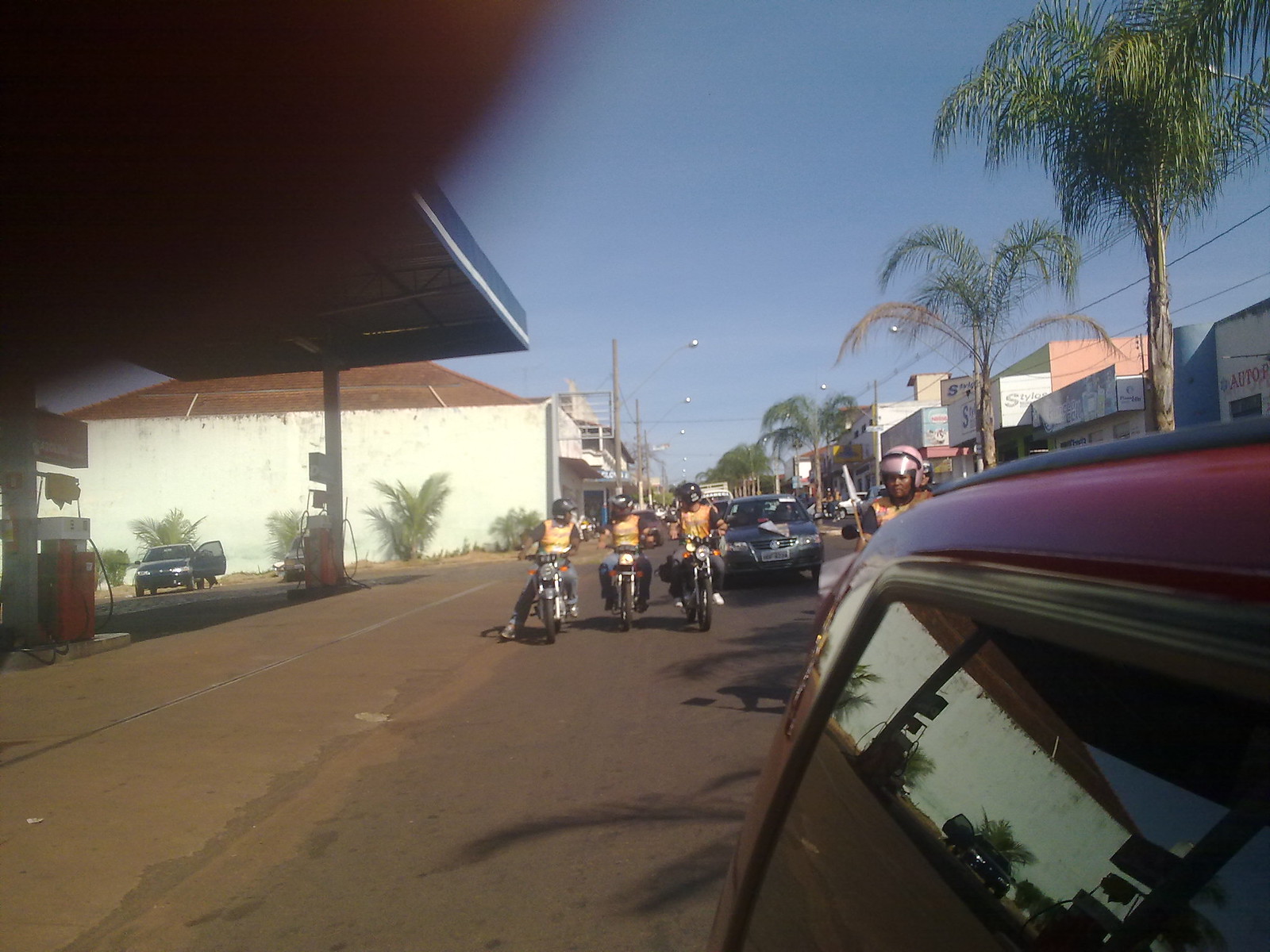In this outdoor, horizontally-aligned rectangular photo, we see a street scene with various vehicles and buildings. In the lower right corner is the rear window of a red car, reflecting a gas station to the left. The gas station features two red pumps, a car with an open door, and a white building with a brown roof. Prominently, four motorcyclists are riding down the middle of the road, all wearing yellow vests. Three of them have black helmets, while the fourth, slightly ahead and obscured by the red car, possibly has a silver helmet. Directly behind the motorcyclists is an older, gray sedan. To the right are several older buildings with trees lined up along the street. The left side also shows more buildings and greenery in front of the white building by the gas station. The blue sky provides a backdrop, and the asphalt street is visible under the vehicles.